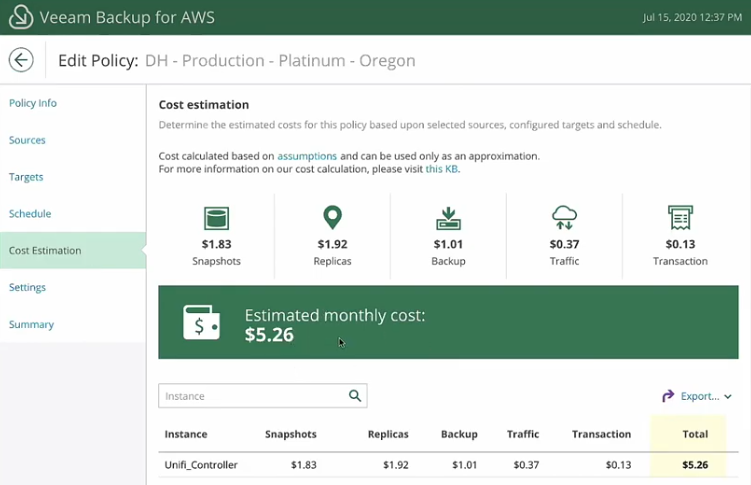Screenshot of the Veeam website on July 15th, 2020, at 12:37 PM, displaying the Cost Estimation submenu under the Edit Policy section for DH Production in Platinum, Oregon. The Veeam logo, spelled V-E-E-A-M, is prominently displayed in white text on a green background. The cost estimation section contains a description stating, "Determine the estimated cost for this policy based upon selected sources, configured targets, and schedule." It further notes that the costs are calculated based on assumptions and should only be used as an approximation. A hyperlink labeled "this KB" in light blue text provides additional information on cost calculation. Below this explanation are icons representing various categories, from left to right: Snapshots, Replicas, Backup, Traffic, and Transaction. Sidebar menus are visible on the left, with the current selection being Cost Estimation.